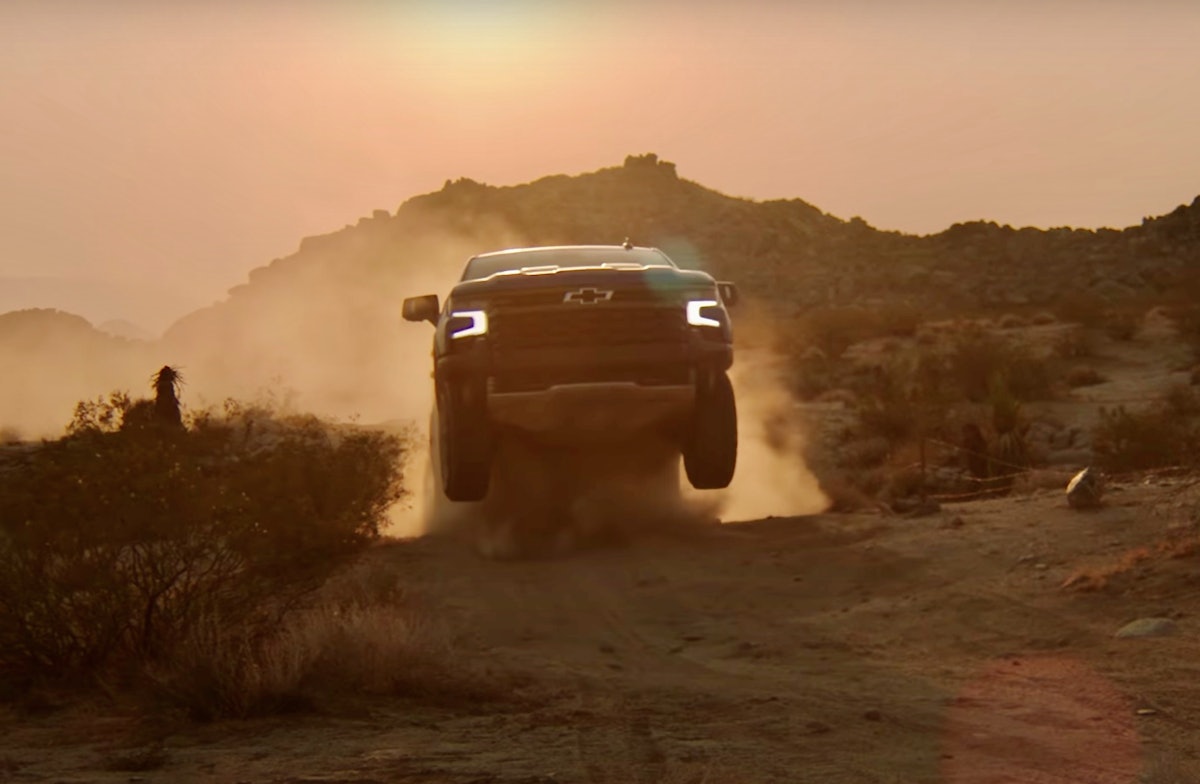In this vivid outdoor scene, set in what appears to be an arid desert, a truck can be seen leaping off a rugged dirt trail, its wheels airborne and leaving a cloud of dust in its wake. The landscape has a pronounced brown tint, with parched soil underfoot and scattered rocks dotting the ground. Dried-up, brown vegetation punctuates the scene on both sides, giving a sense of the harsh, dry conditions. In the background, a range of mountains stretches across the horizon beneath a clear sky. The sun is visible in the upper middle to left area, casting a bright, warm light over the arid terrain.